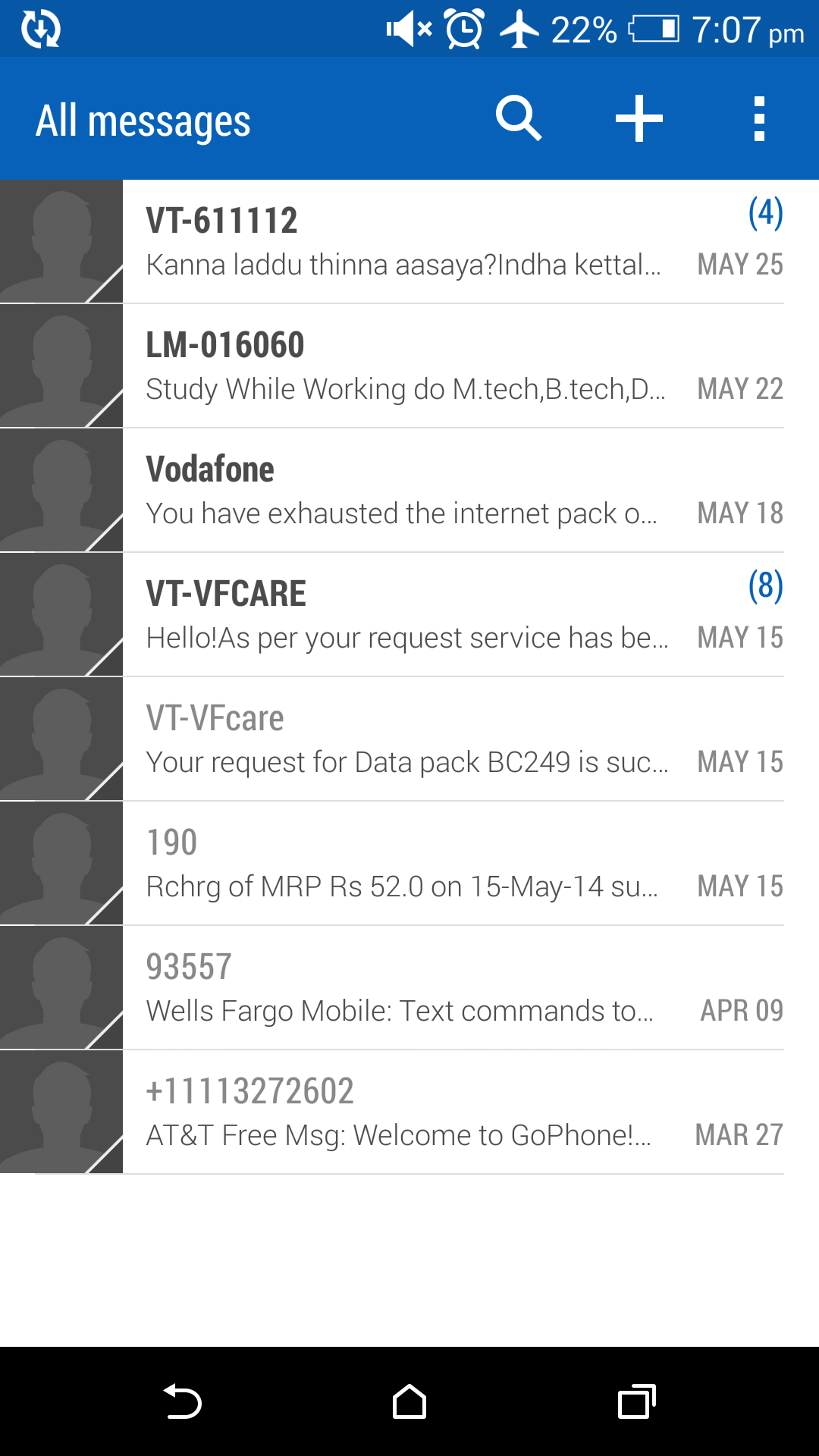The image appears to be a screenshot of a mobile phone interface. At the top of the screen, there's a blue bar, indicating the title "All Messages," with a circular reload icon featuring an arrow pointing downward. Just below this are additional elements: a search icon resembling a magnifying glass, a plus sign icon, and three vertical dots lined up for more options.

Above the blue bar, the status bar displays multiple icons: a muted microphone with an "X," a small clock symbolizing the current time, and an airplane icon showing the phone is in airplane mode. The battery indicator reads 22%, next to the time, which is shown as 7:07 p.m.

The main section of the screen shows a list of messages. There are eight contact icons, all blacked out, aligned vertically. Beside each icon are snippets of text indicating messages, including words and numbers, alongside dates on the far right. Some of these entries have numbers above them, likely indicating unread messages or notifications.

At the bottom of the screen, there's a blank white section, below which lies a black navigation bar. This bar includes a left-facing arrow for back navigation, a house icon for the home screen, and a tab icon representing multiple open tabs or windows.